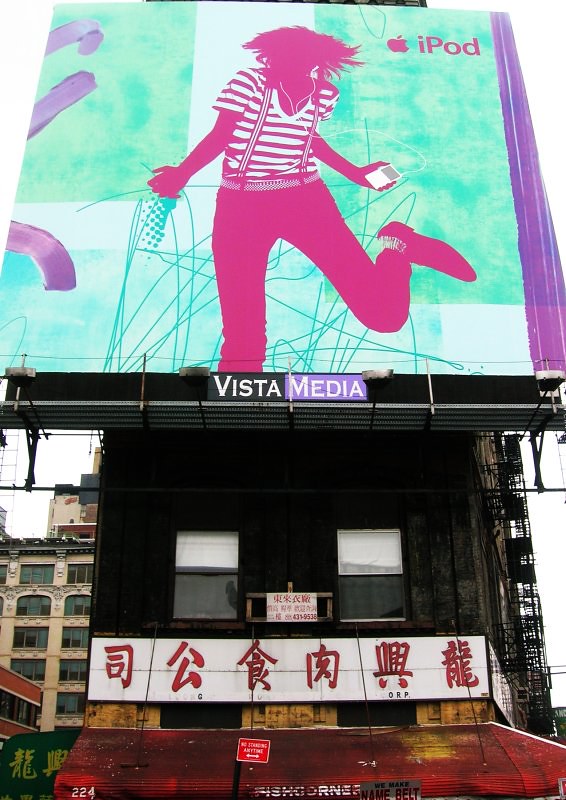An array of advertising hoardings tops a series of buildings in an Asian city, featuring prominent Chinese or Japanese characters in red against a white background, indicative of the region's linguistic heritage. Among these metallic structures, an eye-catching advert for iPod stands out. The advertisement consists of a turquoise background bordered by purple, showcasing a dynamic, magenta-colored silhouette of a dancing figure. The figure, with wild hair, is dressed in magenta shoes and trousers, paired with a striped shirt. Their exuberant dance seemingly resonates to the rhythms of their iPod, encapsulating energy and movement.